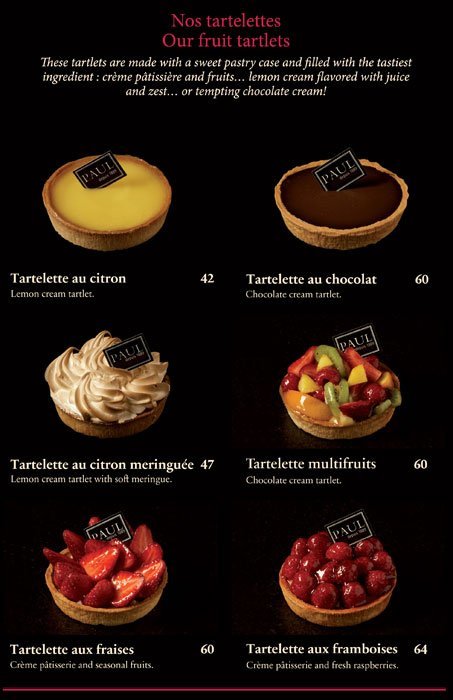The image features a striking pastry menu set against a black background, with text in both pink and white. At the top, "Nos Tartalettas" (Our Fruit Tartlets) is written in pink, while a detailed description in white text beneath it explains that these tartlets are made with a sweet pastry case filled with the tastiest ingredients, including crème pâtissière, fruits, lemon cream flavored with juice and zest, and tempting chocolate cream.

Arranged in two columns and three rows, the professionally photographed images of the tartlets are showcased. The top left image is labeled "Tartelette au Citron" (Lemon Cream Tartlet), followed by "Tartelette au Chocolat" (Chocolate Cream Tartlet) on the top right. In the middle row, the left side features the "Tartelette au Citron Meringue" (Lemon Cream Tartlet with Soft Meringue), while the right side displays the "Tartelette Multi-Frutis" (Multi-Fruit Tartlet). The bottom left showcases the "Tartelette aux Fraises" (Strawberry Tartlet), and finally, the bottom right presents the "Tartelette aux Framboises" (Raspberry Tartlet). Each tartlet is meticulously detailed, emphasizing different flavors and ingredients, such as crème patisserie, seasonal fruits, and French raspberries. This visually striking menu captures both the elegance and delectable variety of the tartlets offered.